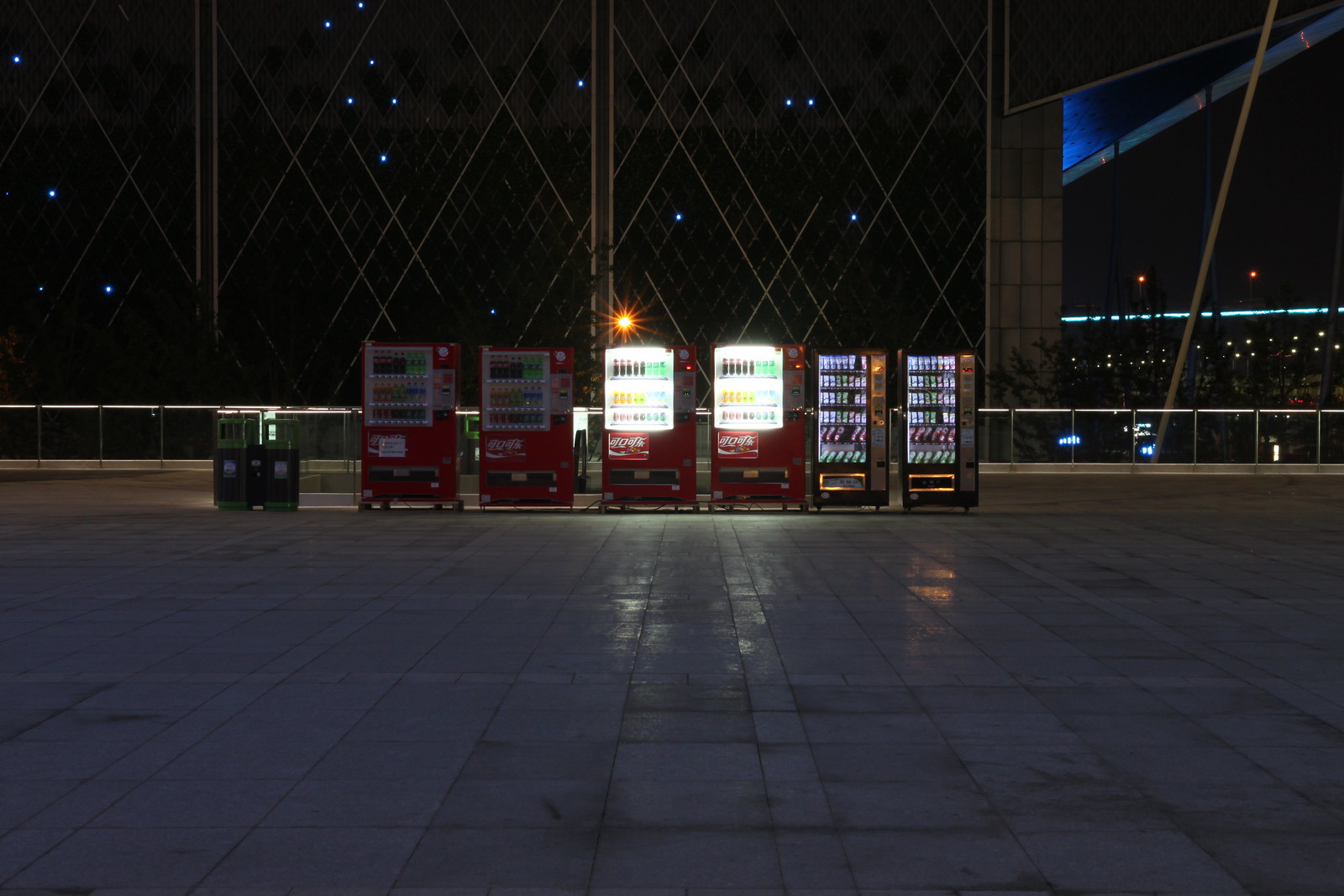This is a detailed nighttime scene showcasing six vending machines arranged on a wide light gray stone-paved walkway, likely situated on an elevated bridge or rooftop. The foreground features two green and gray recycling receptacles on the left. The vending machines, centered in the image, are illuminated against a backdrop of cityscape lights.

Four identical red Coca-Cola beverage vending machines stand prominently, with the middle two brightly lit, revealing bottles of soda inside. Flanking them on the right are two metallic silver and black vending machines, also illuminated, containing an assortment of snacks.

In the immediate background, a steel barrier with a see-through structure suggests the elevated nature of this location. Beyond this barrier, the distant cityscape glows with bright lights attached to towering buildings. Adjacent to the vending machines is a side of a building adorned with diamond-shaped windows and a scattering of bluish-colored neon lights, probably reflecting from adjacent structures.